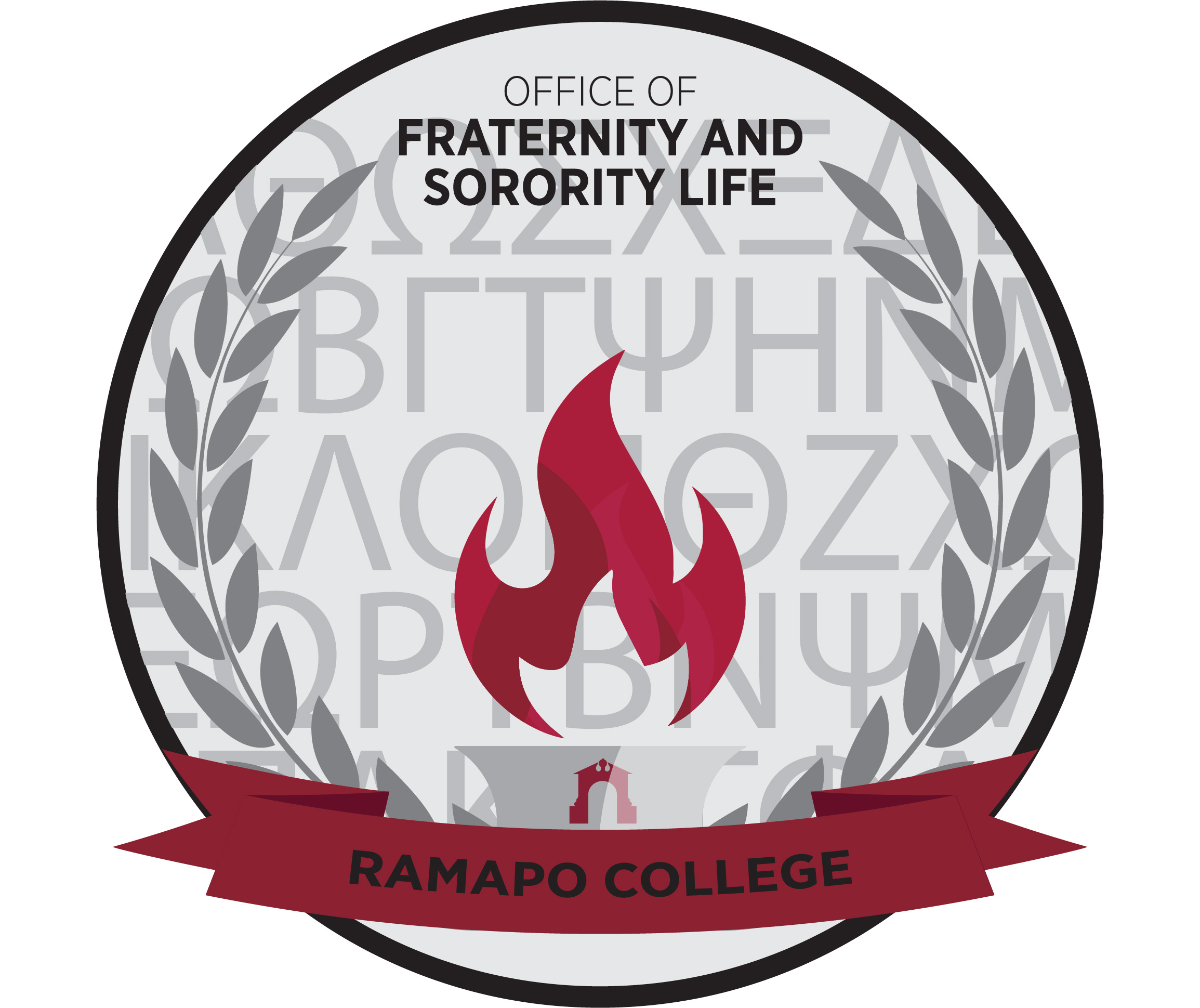This digital graphic features the emblem for Ramapo College's Office of Fraternity and Sorority Life. It is a circular design with a black outer rim. At the top of the circle, the text reads "Office of Fraternity and Sorority Life" in black. The centerpiece of the emblem prominently displays a red flame, flanked by gray leaves on either side. At the bottom of the circle, there's a red ribbon with "Ramapo College" inscribed on it. Additionally, there are Greek letters in gray, positioned as a kind of watermark behind the central flame design. The emblem overall has a black lining with no specific background, emphasizing its use as a digital logo.